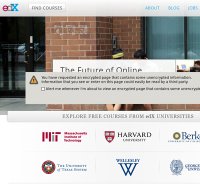The image captures a web page featuring the edX platform. In the top left corner, the edX logo stands out with the 'e' in red, 'd' in green, and 'x' in blue. The page seems to offer information about courses, though some text appears hazy and indistinct. Dominating the central part of the image is an error message, marked by a yellow caution sign with an exclamation point, set against a gray background. The message indicates that the user has encountered an issue related to a requested email, but the full text is not legible.

Behind the error message, the background reveals an image of a brick building, likely a college, given the faintly visible text hinting at online features. The building features metal doors, and reflections of cars are visible. To the right, windows and two students seated are partially visible. The bottom section of the page prominently displays logos and names of various institutions including Harvard, Berkeley, Wesley (identified by two Vs forming a W), MIT, and an unidentified college.

Overall, the web page presents a blend of educational branding and a technical hiccup, overlaid on a collegiate setting.